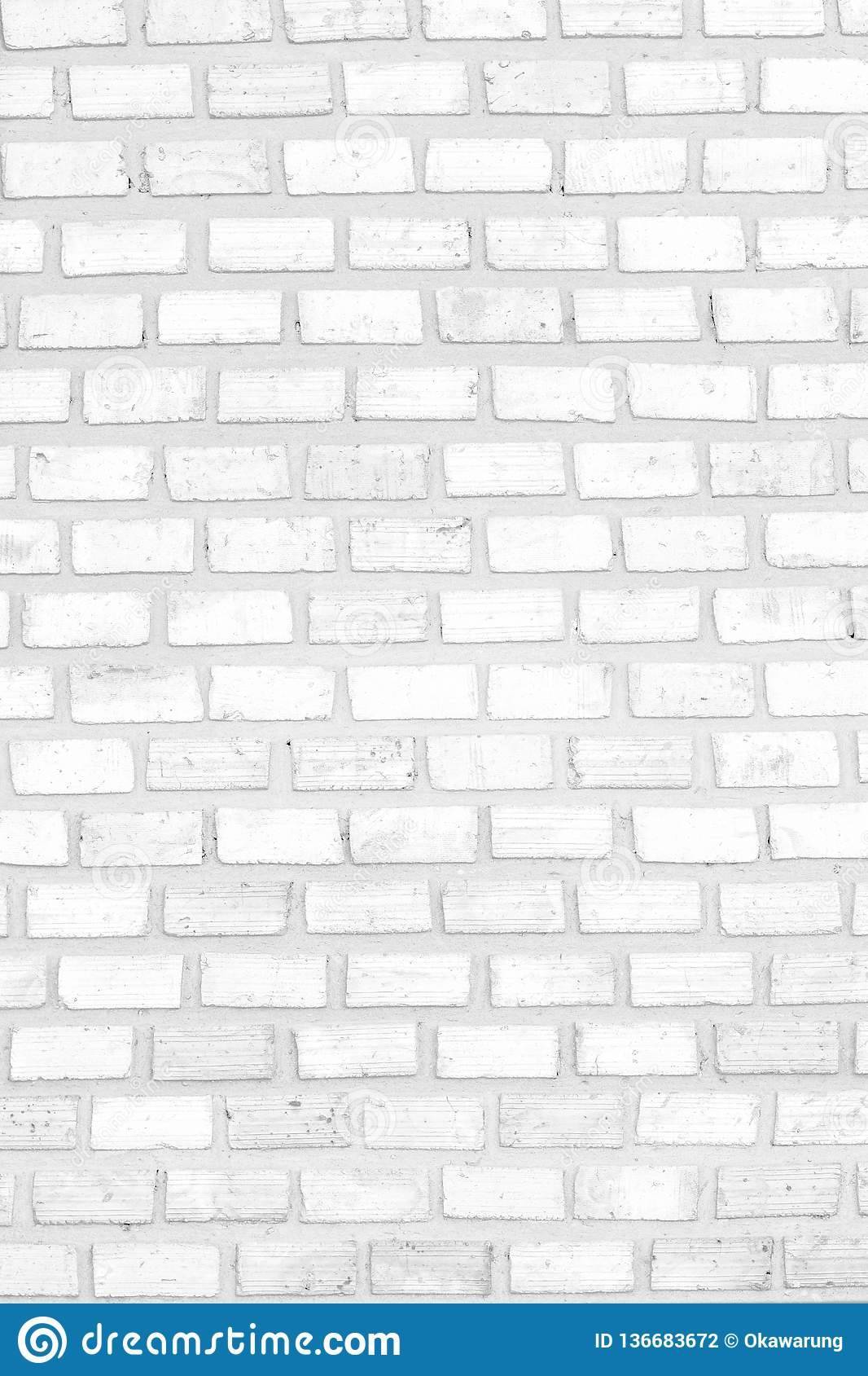The image showcases a rectangular, vertically oriented white brick wall, appearing approximately six inches tall and three inches wide. The bricks, painted white including the grout, exhibit varying degrees of imperfections and lines, lending them a weathered, animated appearance. The thick grout between the bricks enhances their distinctive, irregular look. Scattered throughout the wall are watermarks resembling semi-transparent white swirls, indicative of a digital overlay. At the bottom of the image, a blue footer spans the width, featuring a white swirl on the left beside the text "dreamstime.com." On the right side of the footer, the identification "ID 136683672" is visible, along with a copyright symbol and the name "Okowarone." The repeated presence of the Dreamstime logo and watermark suggest the image is available for sale, potentially as a sample plaster design.